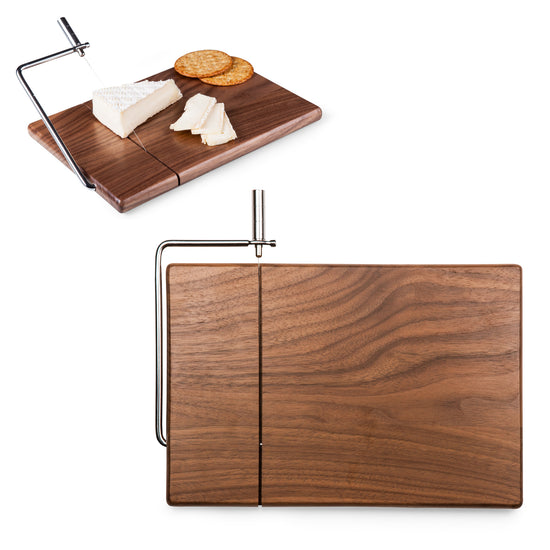This image showcases a wooden charcuterie board with a unique metal slicing mechanism for cheese. The main, larger photo at the bottom depicts a rectangular wooden board laid flat, with a silver metal rod emerging from the left side, arching upwards, and incorporating a heavier vertical rod at a 90-degree angle. This rod assembly, designed for slicing, is equipped with a white string that suggests cutting functionality. Resting on the wooden board is a wedge of brie or camembert cheese, accompanied by three to four neatly cut slices of the same cheese and two round crackers positioned at the upper edge.

The smaller image, inset in the top-left corner, offers a closer look at the operation of the board and metal contraption. The board is tilted, emphasizing the alignment of the rod and string designed to interactively slice the cheese. The display further highlights the tidily cut brie slices and the accompanying crackers, modeling the board’s use. The arrangement and repeated emphasis on the brie slices and the intricate metal rod suggest that this is an advertisement for a specialized charcuterie serving and slicing board, showcasing its functionality and elegant presentation.